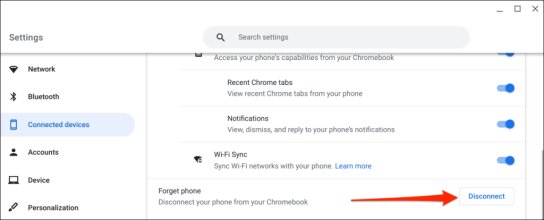This screenshot displays a settings page on a computer, characterized by a predominantly white background. 

In the upper section, a gray box is labeled "Settings" and "Search Settings." On the left-hand side, a vertically aligned menu is present, featuring several options. The first option, "Network," is in bold black text. Below it, "Bluetooth & Connected Devices" is highlighted within a blue box, indicating it is currently selected. Further down the menu, options for "Accounts" and "Device Personalization" are listed.

On the right-hand side, the content relates to integrating your phone's functionalities with your Chromebook. The text begins with "Access your phone's capabilities from your Chromebook," adjacent to which a prominent blue toggle button indicates this feature is enabled.

Below this, several options are listed:
1. "Recent Chrome Tabs" – a blue button toggle here shows this feature is active, along with a description stating, "View recent Chrome tabs from your phone."
2. "Notification" – this section explains the abilities to "view, dismiss, and reply to your phone's notifications."
3. "Wi-Fi Sync" – stating, "Sync Wi-Fi networks with your phone," and a "Learn more" link in blue text. The feature is also active as indicated by a blue toggle button.

At the bottom, an option titled "Forget Phone" offers to "disconnect your phone from your Chromebook." This is highlighted by a large red arrow pointing to the word "Disconnect," which is presented in blue text.